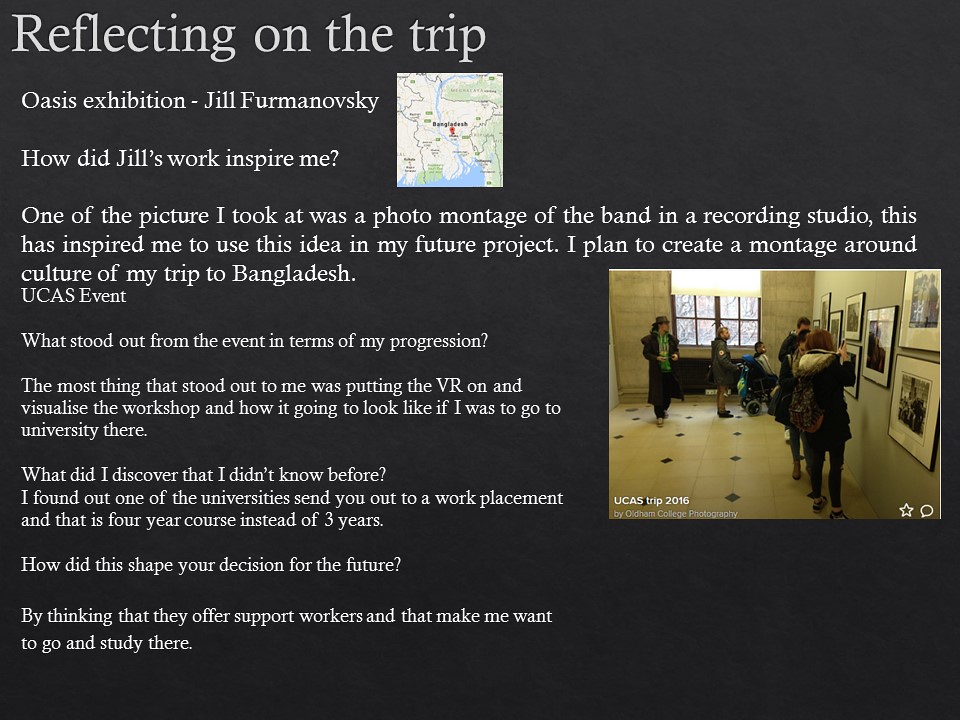The image is a detailed digital presentation slide with a predominantly black background and white text, complemented by photographs. At the top, in large white font, it reads "Reflecting on the Trip, Oasis Exhibition, Jill Furmanovsky." Below this, the caption "How did Jill's work inspire me?" is posed.

On the right side, there's a small map of Bangladesh with a red dot marking a specific location. Adjacent to the map, a paragraph outlines the inspiration drawn from Jill Furmanovsky's photo montage of a band in a recording studio. This inspired the creator to plan a similar montage focused on the culture experienced during a trip to Bangladesh and a UCAS event in the UK. 

To the right of this paragraph, there's a photo featuring six individuals, including a man in a wheelchair, examining framed pictures on a gray wall, reminiscent of an art gallery setting with a large window to the left.

At the bottom left, another caption reads, "UCAS Trip 2016 by Oldham College Photography." A star and a speech bubble icon are placed at the bottom right of the slide.

On the left side, in smaller white text, the slide notes, "What stood out for my event in progress?" It recounts the key highlight as the VR visualization workshop which simulated university attendance. Additionally, the narrative explains discovering that some universities offer a four-year course with work placements, shaping the creator's decision to pursue further studies supported by the amenities provided.